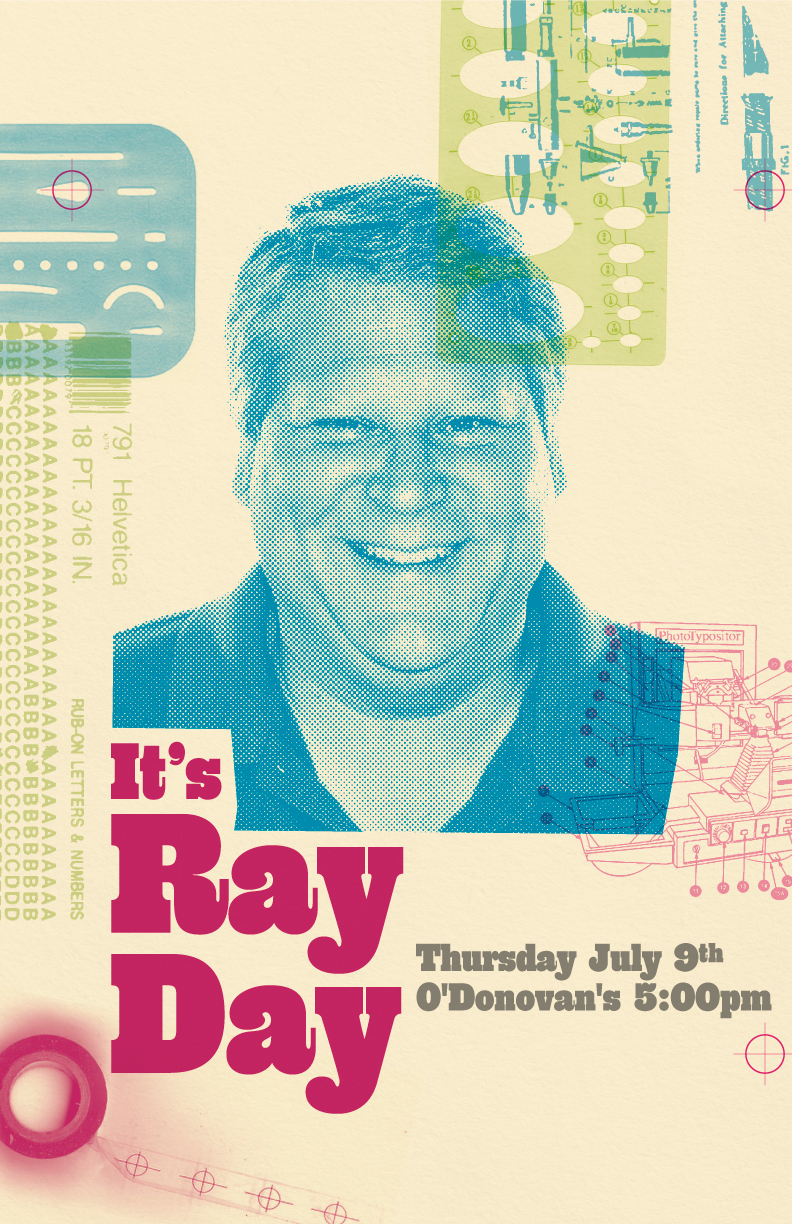This tall rectangular poster advertisement features a detailed collage with a beige background. Prominently displayed in the center is a blue, somewhat pixelated photograph of a smiling man, visible from the shoulders up. He has short brown hair with highlights, is slightly overweight with a double chin, and is dressed in a dark, collared button-up shirt with the top button undone.

Directly to the left of the man's photo, in bright pink fancy font, reads "It's Ray Day," while to the right, in gray text, it states "Thursday, July 9th, O'Donovan's, 5 p.m."

Adding to the intricate design are various artist tools and technical drawing elements scattered across the background. These include templates with rounded circles, dots, lines, and curves, as well as shapes resembling cones and other geometric figures. A transparent light green ruler with several ovals cut out extends from the top right side, and a transparent blue tracing object is visible from the top left. Among these overlays, there are technical drawings or patent-like illustrations, including detailed diagrams and schematic images, possibly of architectural or aeronautical origin. One notable feature is a circular element resembling a rifle scope with crosshairs situated below the event details. Text in small print also specifies precise measurements such as "18.3 sixteenth of an inch" and alphanumeric codes like "A BBB CCC," further enhancing the collage's technical aesthetic.